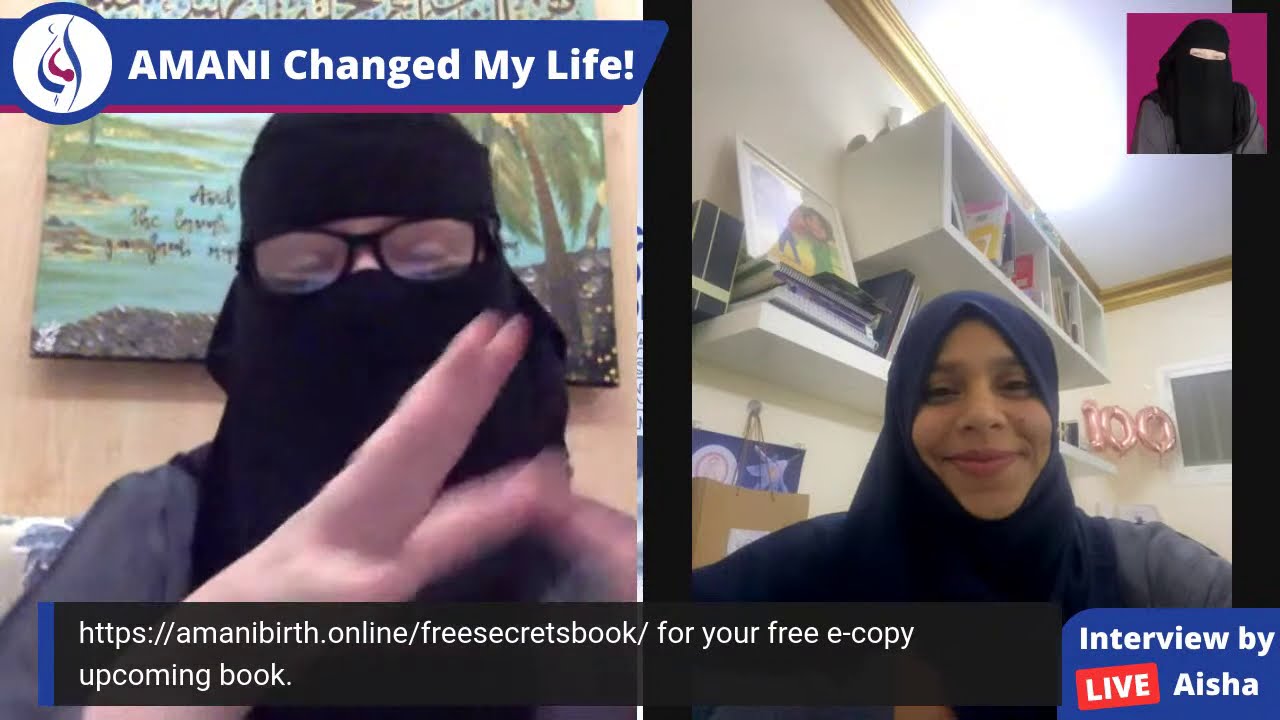The image shows a live video call between two women, displayed side-by-side on a split screen. At the top left of the image, there's a blue banner with a white interior circle that features a symbolic depiction of a pregnant woman, accompanied by pink shapes representing a baby. The banner includes the title "AMANI CHANGED MY LIFE!" in bold white font. In the bottom right corner, a smaller red box with the word "LIVE" indicates the broadcast status, accompanied by the phrase "interview by Aisha."

The woman on the left is dressed in a black head covering that conceals her entire face except for her eyes, and she's wearing glasses. Her clothing appears to be grey. The woman on the right is smiling and looks happy; her head is covered with a dark blue headscarf, but her face is exposed. She is also wearing grey clothing and is seated in front of shelves filled with books and other objects. At the bottom left of the image, an opaque black banner features the link "https://amanibirth.online" along with a mention of a free e-copy of an upcoming book titled "Free Secrets Book."